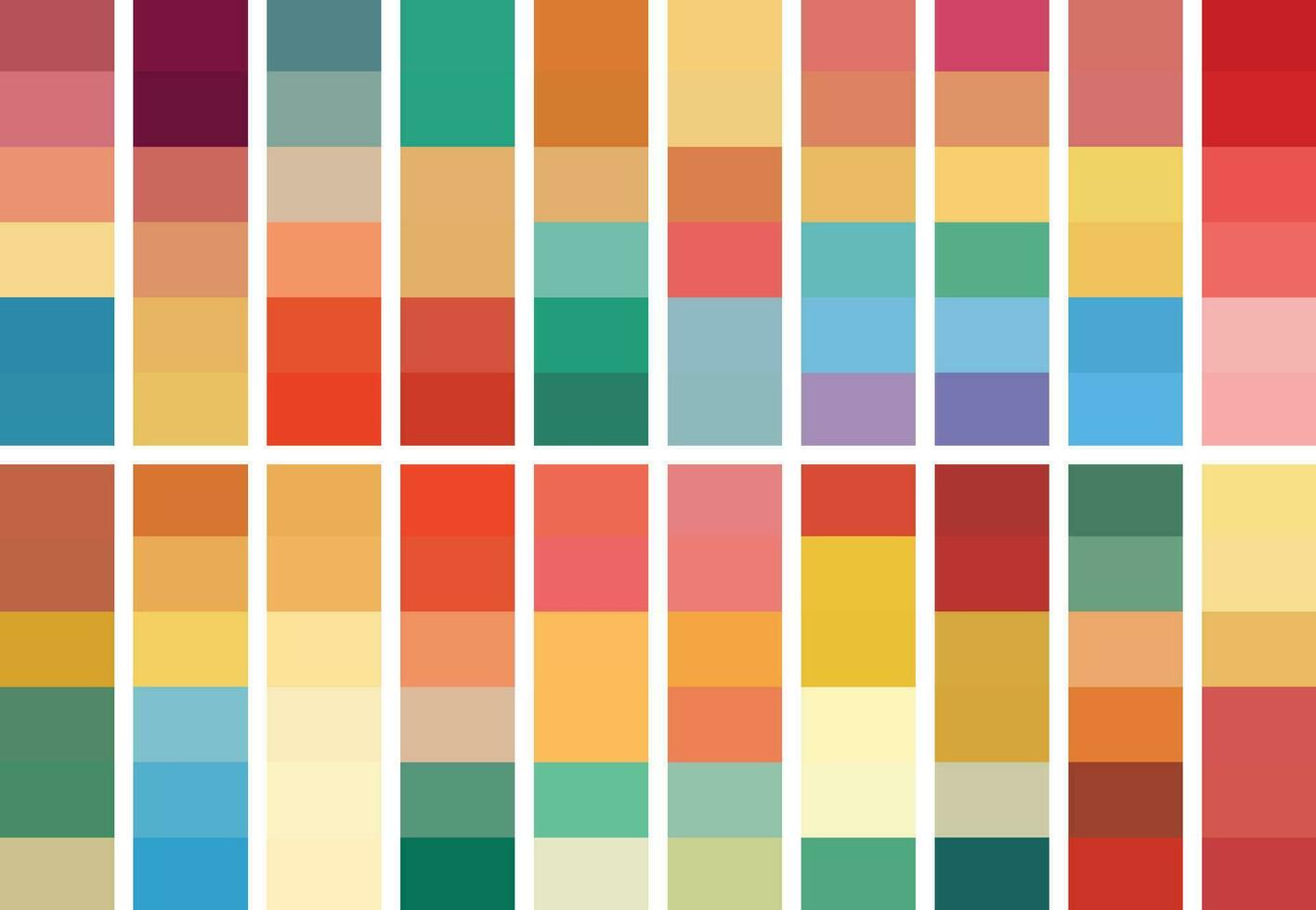The image depicts 20 meticulously arranged rectangles, 10 on the top row and 10 on the bottom, each resembling paint sample cards. Every rectangle is divided into six distinct color sections, presenting a striking variety of hues including shades of red, orange, yellow, green, blue, pink, tan, brown, gray, and white. The colors are predominantly warm and bright, though some are slightly muted, creating an interesting combination that suggests a southwestern style. Despite some colors being subtly different to the point of appearing almost indistinguishable, the overall palette maintains a vibrant diversity. The alignment and color choices hint at a potential AI generation, underscoring the unique, almost nonsensical micro-variations in color that provide an intriguing visual experience.